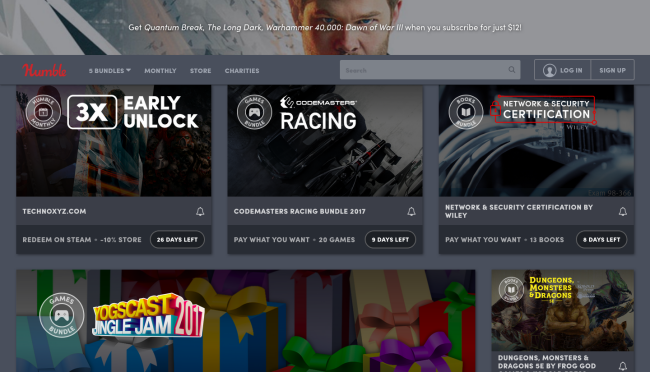This is a detailed screenshot of the Humble site interface. In the top left corner, a gray bar hosts the bold red "Humble" logo. Dominating the upper center of the image is a close-up of a man with piercing eyes staring directly at the camera. White text overlaid across the bridge of his nose reads: "Get Quantum Break, The Long Dark, Warhammer 40,000, Dawn of War 3 when you subscribe for just $12."

Beneath this central image, a darker gray line spans the width of the page. To the right of the red "Humble" logo, white text labels the site sections: "Bundles," "Monthly," "Store," and "Charities." Adjacent to these sections is a gray search entry box with a magnifying glass icon on the far right. Two rectangular, white-outline buttons are positioned on the far right: the left button features a white circle with a human icon and the text "Login," while the right button reads "Sign Up."

Directly below this dark gray line are three distinct sections. On the left, bold white text declares: "3x Early Unlock, Technics.com, Redeem on Steam." The center section, in bold white, promotes: "Racing, Codemasters Racing Bundle, Pay What You Want, 20 Games." On the far right, outlined in a red square with a padlock icon, white text announces: "Network and Security Certification, Network and Security Certification by Wiley, Pay What You Want."

Beneath these sections, the page background features a large image area. Centrally located within this area is a dual-circle icon with white text reading "Games and Bundle." A white game controller icon is in the center. To the right, the image showcases several gifts wrapped in bold yellow, pink, purple, and green ribbons. In the far right corner, yellow text reads: "Dungeon Monsters and Dragons," with follow-up text at the bottom stating: "Dungeons, Monsters, Dragons SE or 5E by Frog God." 

Lastly, a gray notification bell is positioned in the very bottom right corner.